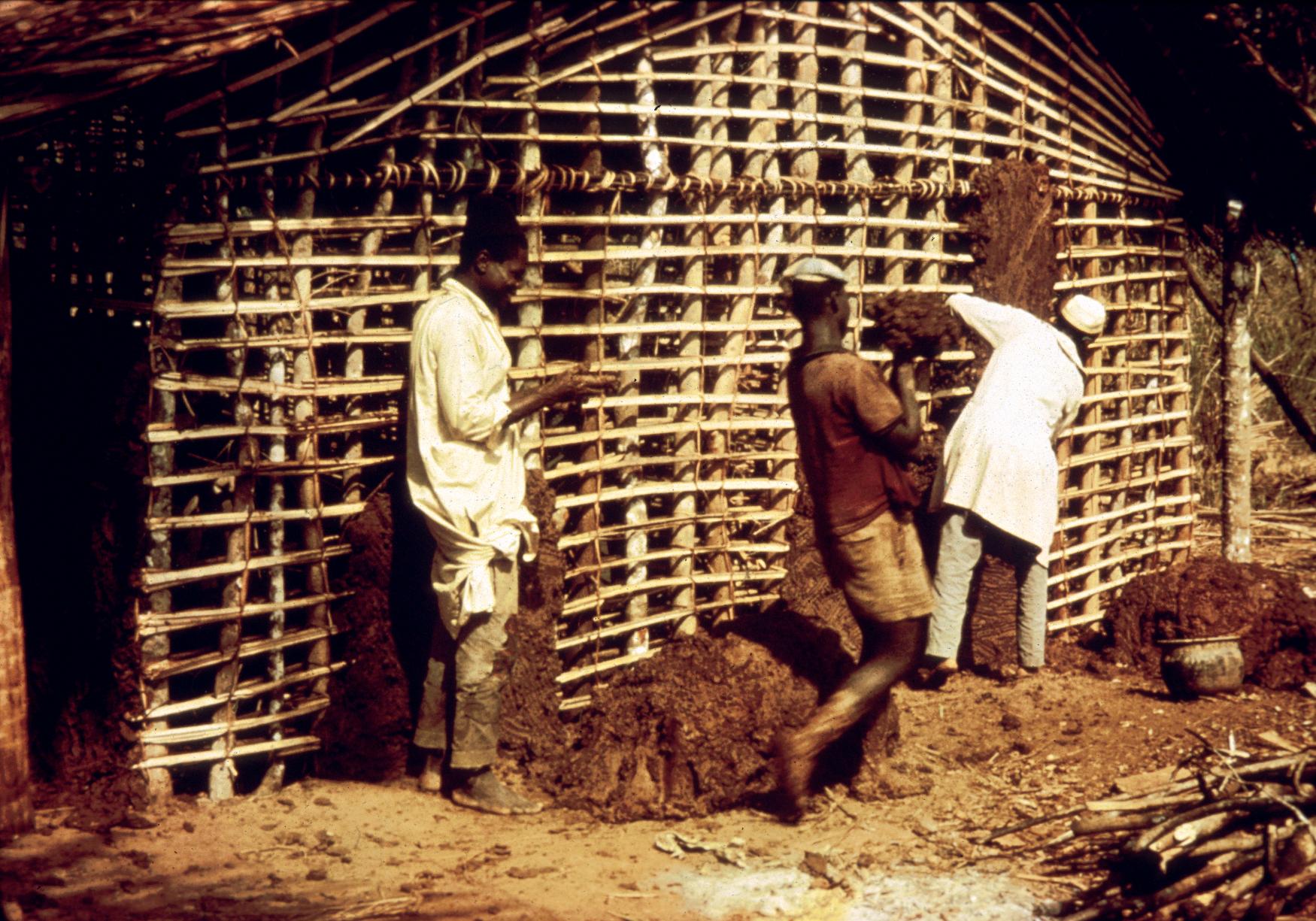In the sepia-toned image, three dark-skinned men are engaged in building a wooden structure, likely a house, using an intricate crisscross pattern of wooden sticks and bamboo. The man on the left, barefoot and wearing a long white shirt with pants, is studying something in his hand. In the center, a barefoot man in a brown short-sleeve shirt and shorts, with mud-caked legs, is carrying a mound of dirt or mud. On the right, another barefoot man, dressed in a reddish-orange top and yellow pants, is applying the mud to the structure. They are all standing in a muddied area surrounded by dirt and sticks, working diligently in front of a skeletal frame of vertically and horizontally aligned light brown branches, topped with a triangular roof of the same material. The overall earthy tones of the photograph evoke a sense of an older, possibly rustic setting.